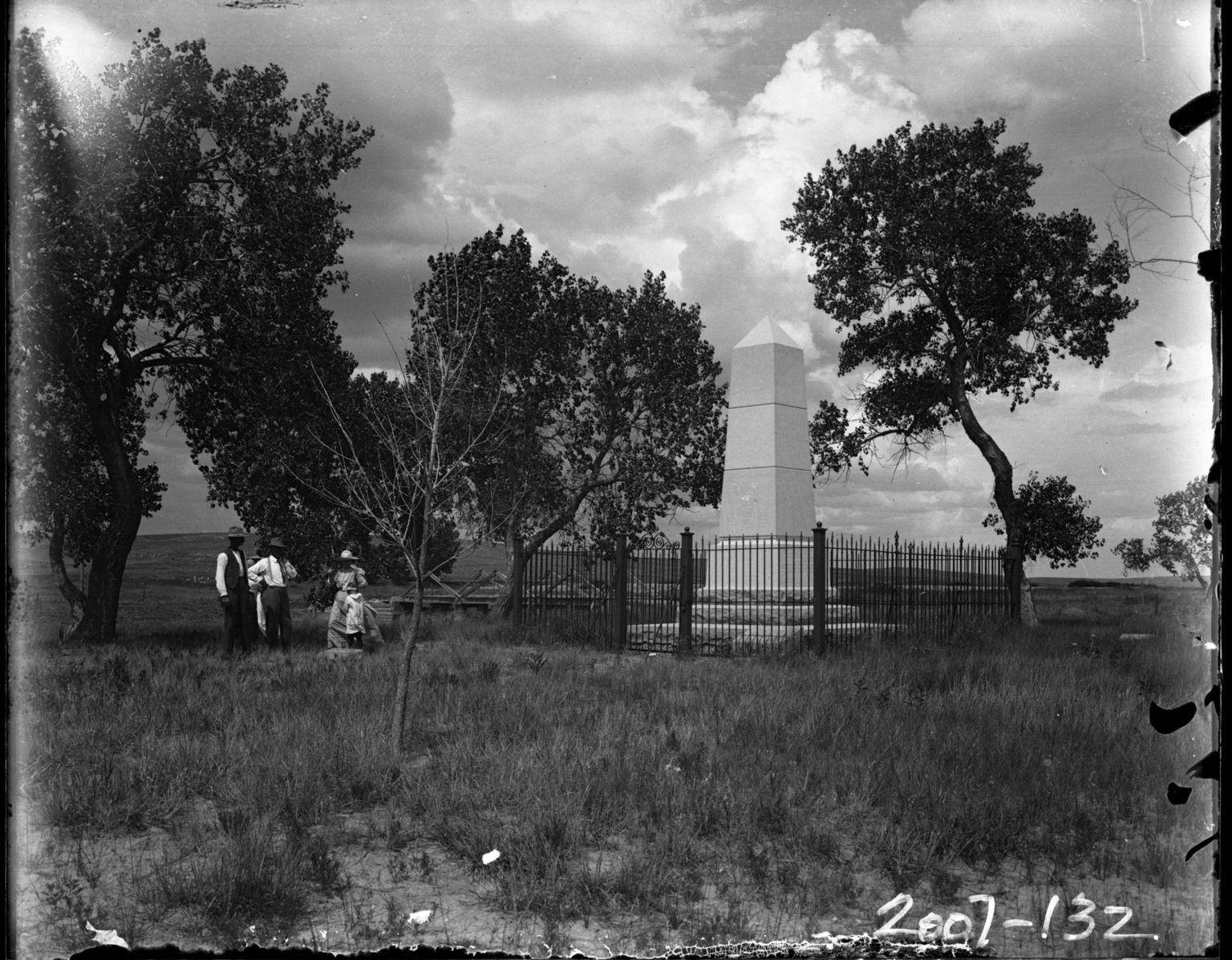This black-and-white photograph, seemingly a scan of an old image, depicts an outdoor scene with a white stone obelisk enclosed by a wrought iron fence, standing prominently in a grassy field. Surrounding the obelisk are multiple trees, casting a serene, somewhat somber atmosphere reminiscent of a cemetery or memorial site. To the left of the monument, three figures, appearing to be African American and dressed in 19th-century attire, stand gazing at the structure. The men are wearing hats, suspenders, white shirts, and dark pants, while the woman is clad in a light-colored dress and a hat. The photograph captures a vast sky filled with large gray clouds, enhancing the historical and contemplative mood. Notably, the image edges are faded and show signs of wear, hinting at its age. In the bottom right corner of the photo, there is an inscription in white text, likely reading "2007-132," although it could be "ZOOL-132."